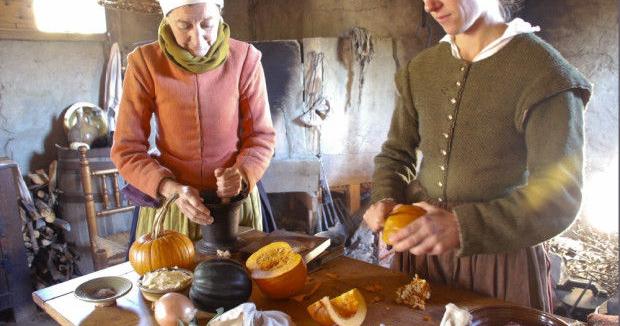In this detailed image, we observe a rustic indoor kitchen setting, resembling a scene from colonial or early 18th-century times, possibly a recreation with actors portraying pioneer people or Puritans. The photograph, longer than it is tall, captures two individuals, likely women, engrossed in preparing various types of squashes on a wooden table. The elderly woman on the left, dressed in a salmon-colored jacket, a green scarf, and a blue and green skirt, meticulously handles the produce. The person on the right, whose head is cut off at the top of the frame, wears a dark green multi-button vest over a long-sleeved green shirt with a white collar, highlighting a task-focused demeanor, probably cutting one of the squashes with a knife.

The table before them is an autumn bounty featuring an assortment of squashes: small, pumpkin-colored ones, a dark green acorn squash, a butternut squash, as well as garlic and onions. The overall atmosphere suggests a harvest or fall time theme, evoking images of early Thanksgiving or Pilgrim times. Kitchen utensils hang on the stone wall behind them, and a wooden chair is placed behind the woman with the salmon-colored jacket. The setting is further enriched by the presence of old whiskey wine barrels, enhancing the ambiance of a bygone era. The individuals are dressed in period-appropriate attire, layering long-sleeved sweaters that button up to their collars and skirts, fitting seamlessly into the historic theme of this modest, yet detail-filled kitchen scene.